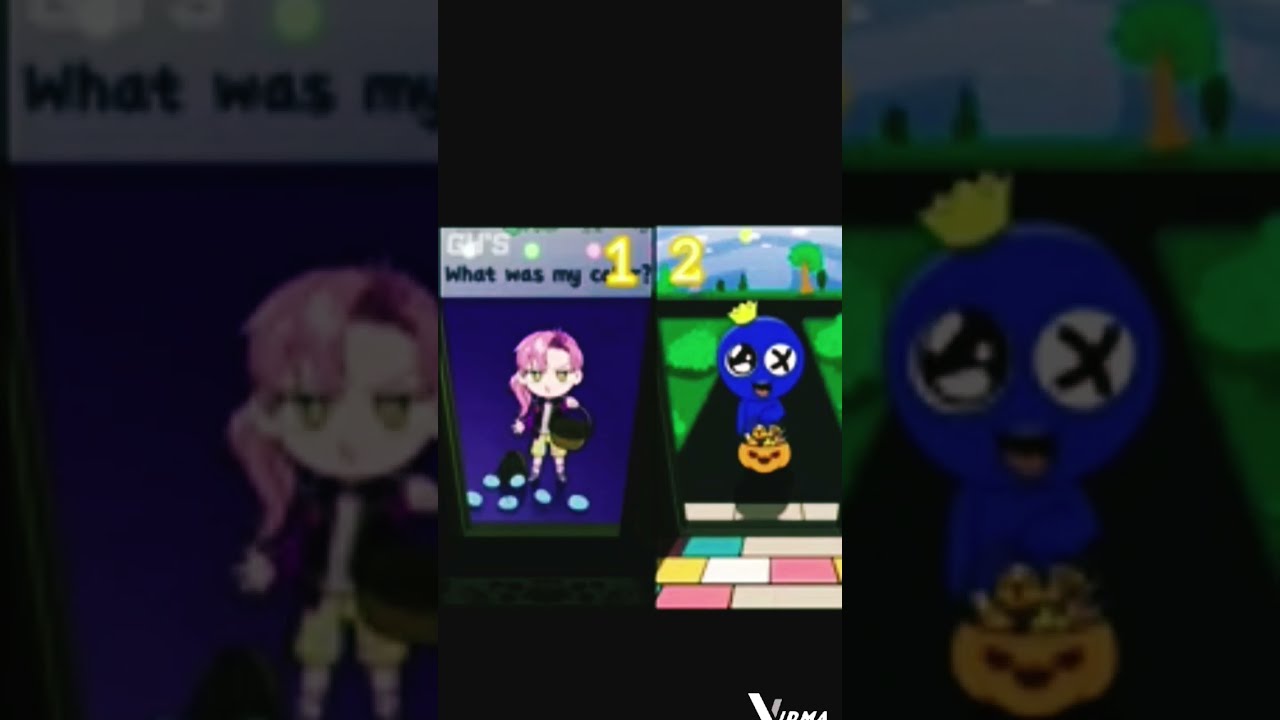The image appears to be a split-screen scene from a cartoonish mobile game, featuring two distinct characters. On the left side, a girl with pink or purple hair and a stern expression stands defiantly against a blue background. She is holding an indiscernible object in her left hand and has a book bag by her feet. Above her, a sentence partially obscured by a yellow number one seems to read, "What was my...". The right half depicts a blue bird-like character with large, quirky eyes—one normal and the other marked with an X. The bird is wearing a small yellow crown, looks happy, and is holding a jack-o'-lantern candy bucket. A number two is displayed above this character. Both characters are centrally positioned within a narrow frame bordered by blurred zoomed-in versions of their own images.